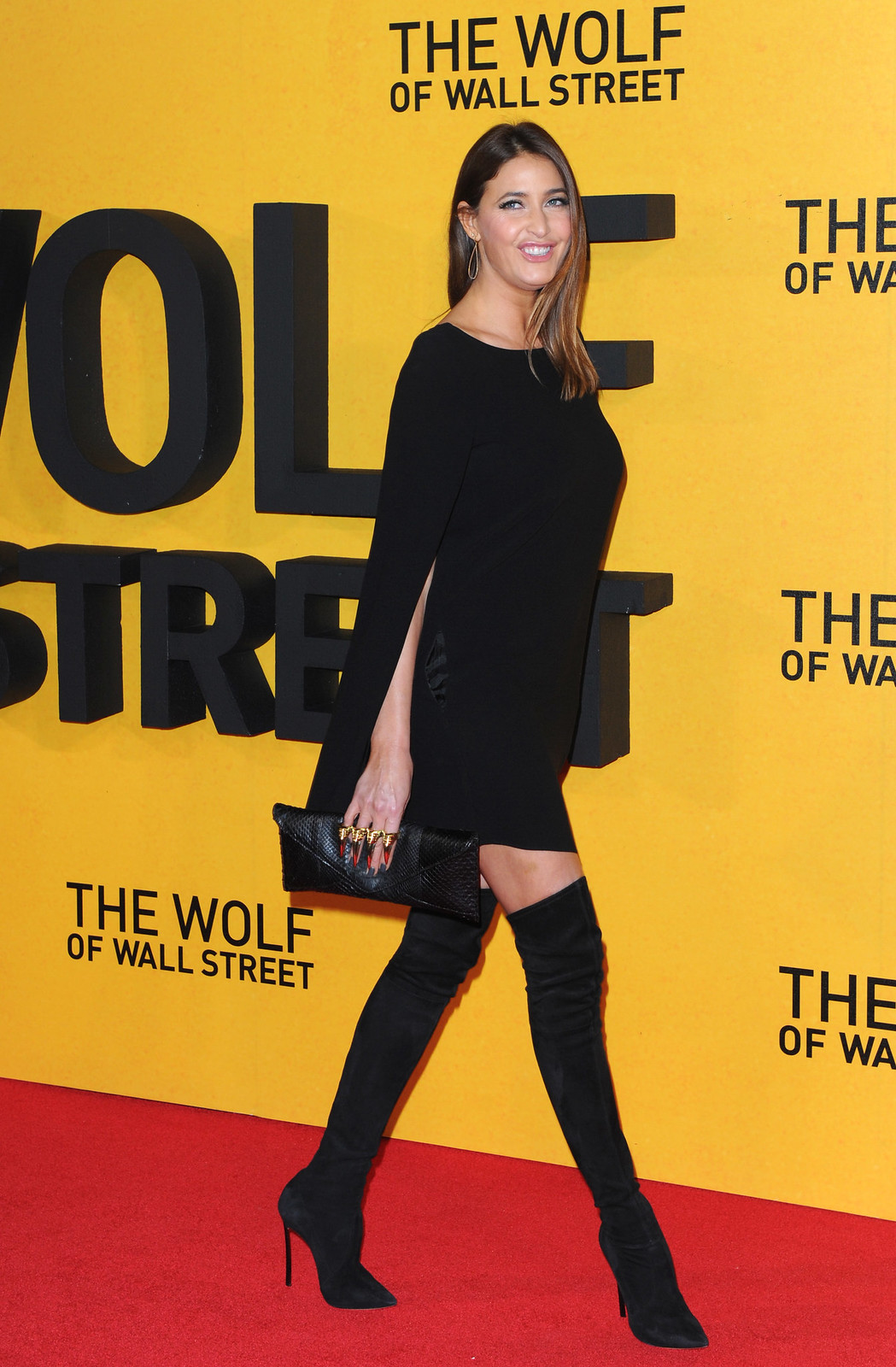The image is a detailed photograph likely taken during the premiere of "The Wolf of Wall Street," indicated by the yellow backdrop repeatedly displaying the movie's title in black print. Captured on a red carpet, the image features Lisa Snowden as she walks past the backdrop. Lisa is smiling directly at the camera, exuding a confident and elegant presence. She wears a short, black dress with a slit that reveals her arm, paired with thigh-high black boots that resemble leggings at the top. Her dirty blonde, shoulder-length hair, accentuated with blonde streaks, is parted on one side. Her ensemble is accessorized with earrings, gold rings, and a small black clutch purse. The overall scene suggests a glamorous event, with Lisa posing intentionally for the photograph on the star-studded red carpet.